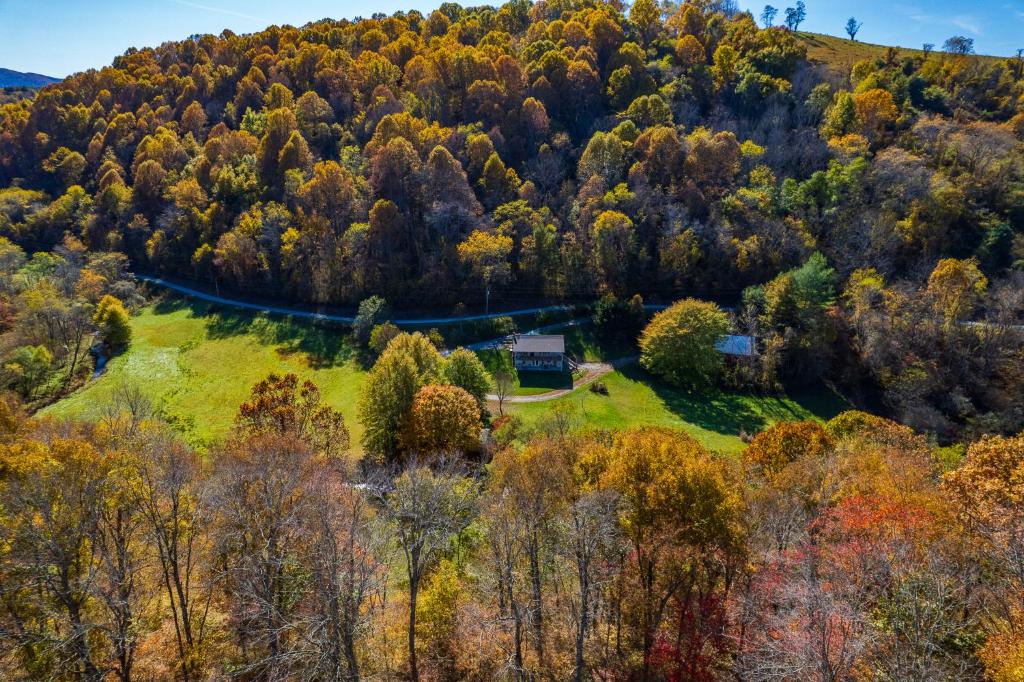This is a detailed aerial shot taken during a clear, sunny day, capturing a scenic landscape in what appears to be fall. At the center of the image, a house sits prominently on a hill, complete with a circular driveway and a hint of a swimming pool peeking out from behind one of the trees. The property is expansive, marked by neatly mowed grass areas surrounded by a lush forest that displays a stunning tapestry of fall colors – vivid greens, brilliant yellows, rich golds, and warm reds. The trees vary in density; some are lush with leaves while others are bare, reflecting the seasonal transition. In the background, rolling hills adorned with a mix of vibrant trees lead up to what appears to be a larger hill or mountain, its top kissing the blue sky. A winding road meanders through the hills, adding to the picturesque quality of this autumnal landscape.